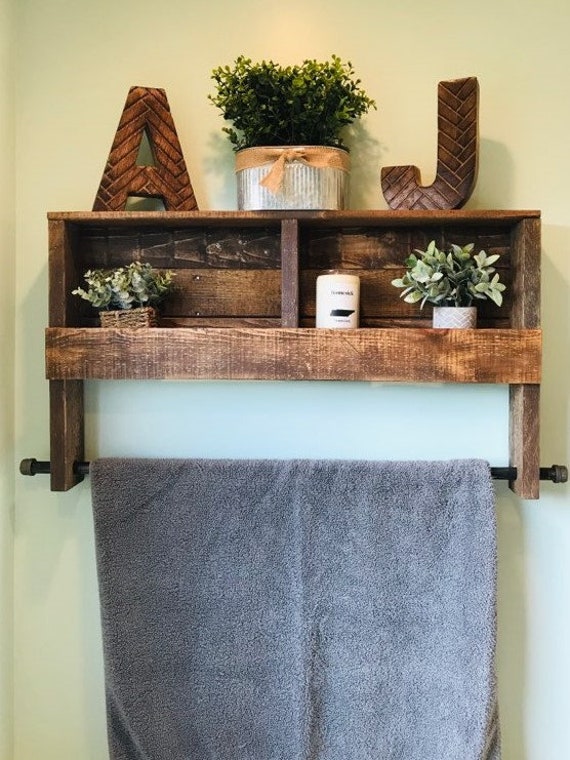The image depicts a detailed setup within a bathroom. At the center of the scene is a rustic wooden shelf shaped like a box with two compartments, adding a touch of vintage charm with its deep brown, weathered finish. On the very top of this shelf stand two sizeable wooden letters, "A" on the left and "J" on the right, both matching the rustic theme. Between these letters is a small gray pot adorned with a light brown to peach-colored ribbon, housing a green shrub.

The shelf is transparent and divided into two sections. The left compartment houses a smaller pot of foliage contained in a wicker basket, while the right compartment holds another pot of greenery placed in a white designed vase, along with a white candle. These sections are separated by a central wooden divider.

Beneath the wooden box shelf, two legs extend down, and a black rod towel rack runs through holes in these legs, neatly supporting a gray and white striped towel. This elegant yet rustic setup combines functionality with aesthetic appeal, making it a charming addition to the bathroom.